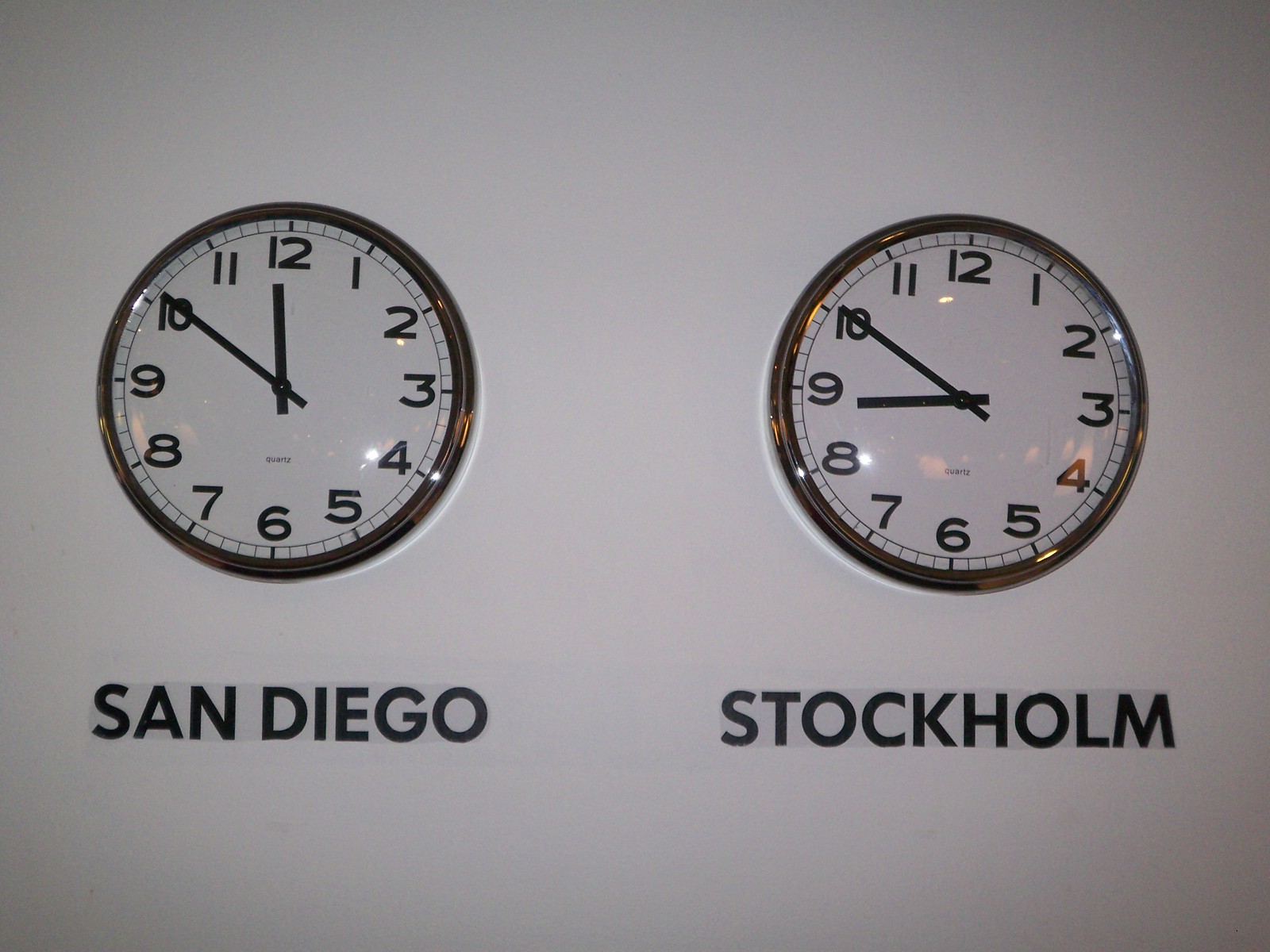In the image, two nearly identical wall clocks are displayed side by side against a wall that appears grayish in the photo but is likely white in reality. Both clocks feature white faces with black hands and regular numerals from 1 to 12, as well as minute markings in between. Each clock has "quartz" written below the center. The clock on the right, labeled "Stockholm," shows the time as 8:50, while the clock on the left, marked "San Diego," shows the time as 11:51. Both clocks are encased in metallic rims that appear more gold than silver. The image is in landscape orientation and is not very well-lit, contributing to the grayish hue of the wall.